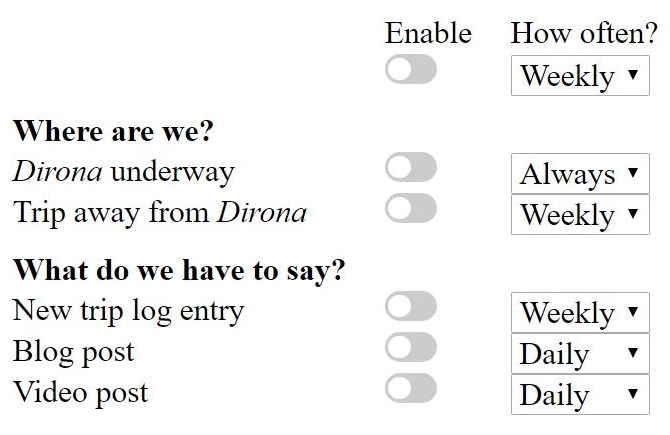**Detailed Caption:**

This image depicts a screenshot of an online interface presented in a landscape rectangular format with a white background, lacking any borders or a header. The layout is divided into three implicit columns, though no grid lines are present to delineate them.

Starting with the widest column on the left, the content is left-justified with no initial entries at the top. The first prominent element is a bold question "Where are we?" followed by two italicized phrases: "Dairana underway" and "Trip away from Dairana". 

Below this section, after a small empty space, another bold question "What do we have to say?" appears. Underneath this are three options: "New trip log entry," "Blog post," and "Video post".

The middle column is headed by the title "Enable". Beneath this are six toggle fields designed as elongated light gray ovals with white circles inside at the left end, indicating they are turned off. The top toggle field aligns with no specific entry in the left column, while the next five correspond to the phrases "Dairana underway," "Blog post," and "Video post" from the left column.

Moving to the right column titled "How often?", there are six landscape-oriented rectangular boxes. Each box contains a dropdown arrow, represented by a small upside-down triangle at the right, signifying additional selectable options. The top field, without a related toggle or entry on the left, displays the word "Weekly". The subsequent boxes align with the corresponding rows from the middle and left columns, displaying "Always," "Weekly," "Weekly," "Daily," and "Daily" respectively.

Summarizing, the interface exhibits a systematic arrangement where the left column presents questions and options, the middle column contains toggles to enable these options, and the right column specifies the frequency settings for the options.